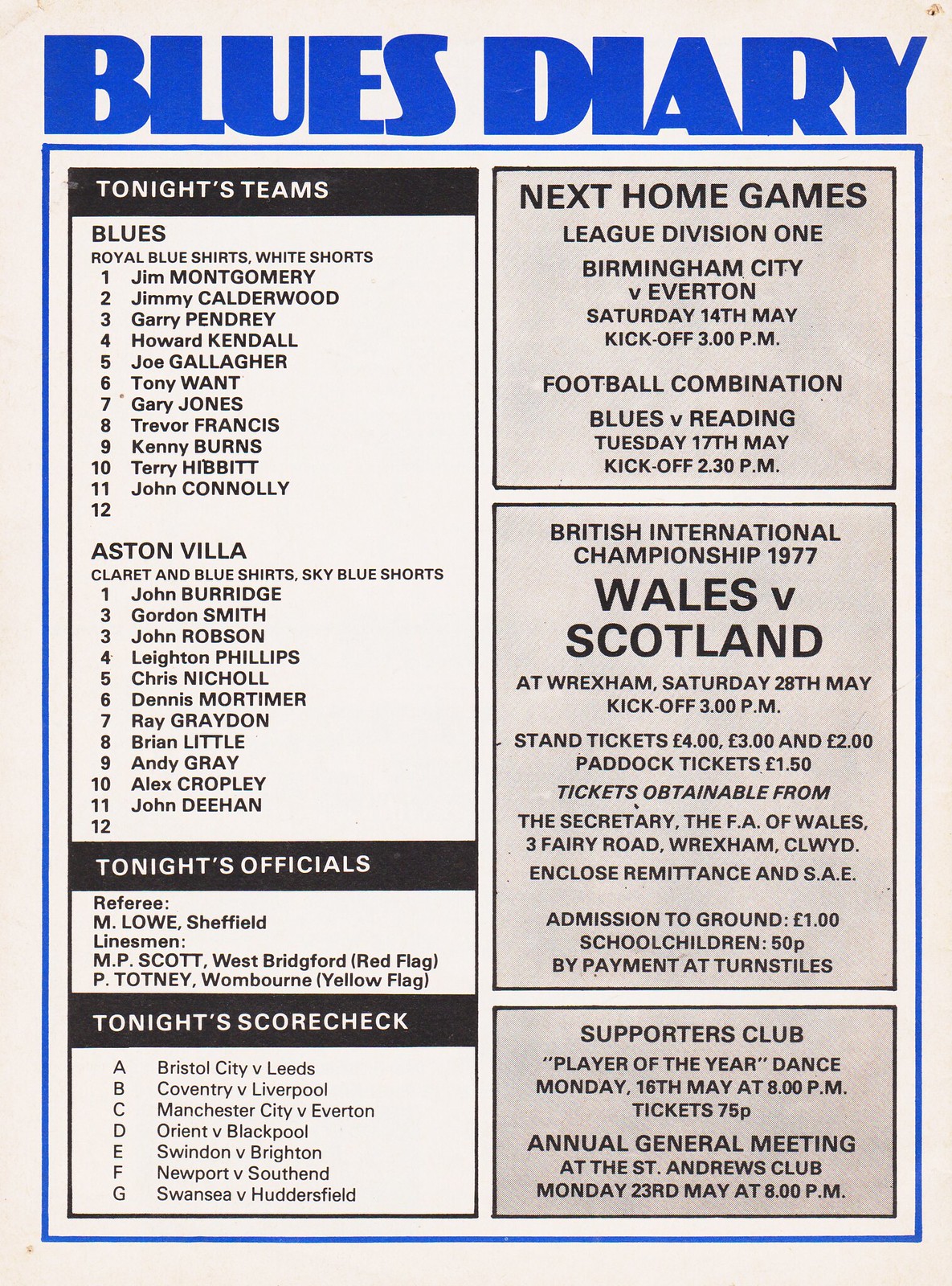The image presents a detailed, sports-themed flyer titled "Blue's Diary" with a blue headline, resembling a magazine page or perhaps a Table of Contents. The flyer is divided into two columns, left and right, each serving distinct sections of information.

On the left side, the column is titled “Tonight’s Teams.” It features two opposing teams: Team Blue, characterized by Royal Blue shirts and white shorts, and Aston Villa with claret and blue shirts paired with sky blue shorts. Each team has a lineup of players numbered from 1 to 11. Below this section is “Tonight’s Officials,” listing the referees, including Amlal Sheffield and linesmen MP Scott and P. Totney. The subsequent section titled “Tonight’s Score Check” covers the scores of various matches from A to G, such as Bristol City versus Leeds, Coventry versus Liverpool, Manchester City versus Everton, Orient versus Blackpool, Swindon versus Brighton, Newport versus Southend, and Swansea versus Huddersfield.

The right column begins with upcoming events under “Next Home Games.” This includes fixtures like the League Division I match between Birmingham City and Everton on Saturday, the 14th of May, with a 3 p.m. kickoff, and the Football Combination game between Blues and Reading on Tuesday, the 17th of May, at 2:30 p.m. The central section announces the British International Championship, 1977, highlighting the Wales versus Scotland match at Wrexham on Saturday, the 28th of May, with a 3 p.m. kickoff. Details include ticket prices ranging from four pounds to one pound, with special rates for school children. Tickets are available from the Secretary, FA of Wales, and can also be purchased at the turnstiles. 

In the bottom right corner, there’s information about the Supporters Club, featuring events like the Player of the Year Dance on Monday, the 16th of May, at 8 p.m., with tickets priced at 75p. It also notes the Annual General Meeting at the St. Andrew's Club on Monday, the 23rd of May, at 8 p.m.